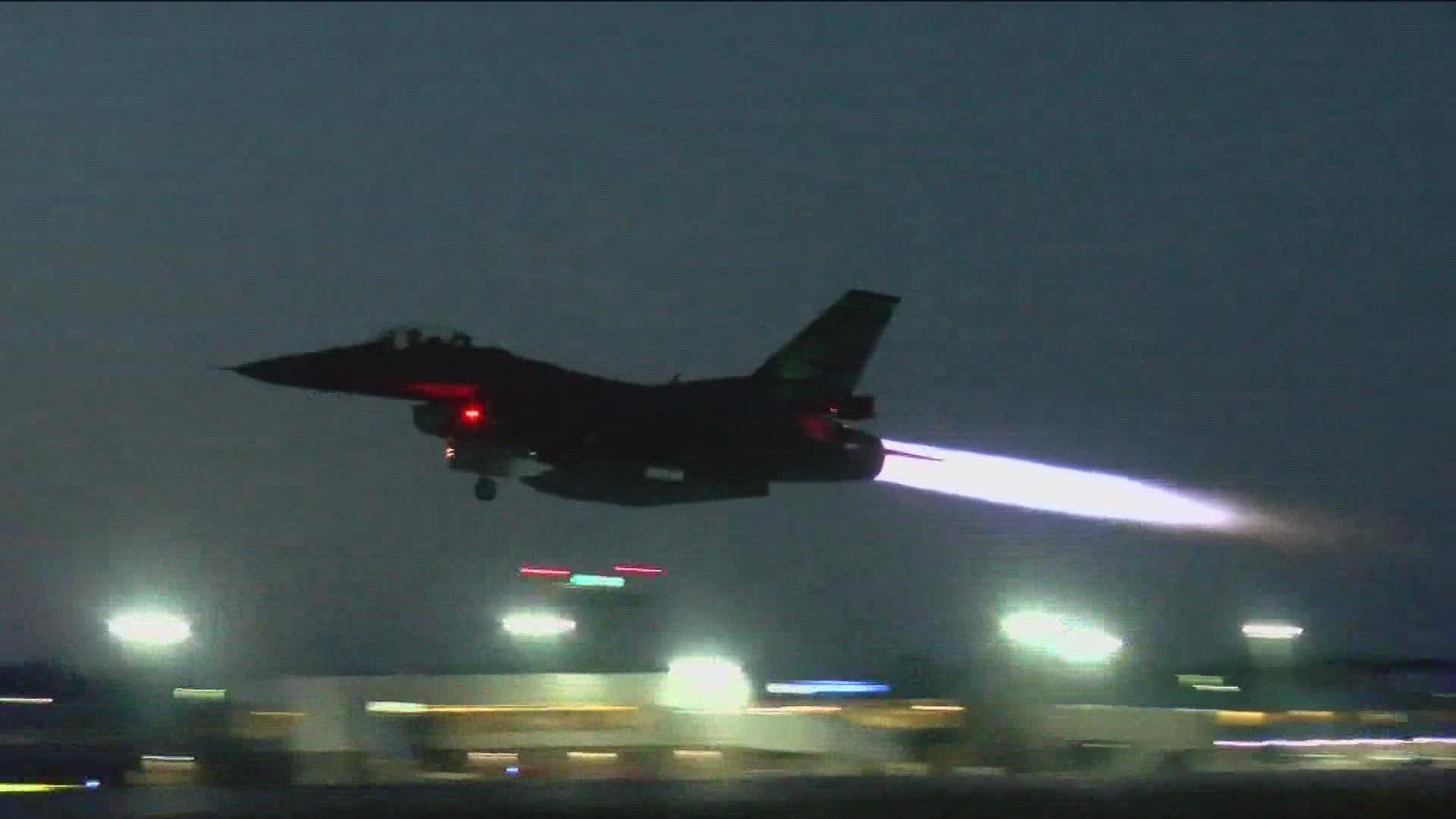This photograph captures the dramatic nighttime takeoff of a military jet, possibly an F-16 or F-15. The jet, silhouetted against a dark, grayish sky, streaks to the left of the frame, characterized by its dark, almost black hue. A vivid burst of white flame trails from its rear exhaust, surrounded by red lighting, emphasizing its speed and power. Beneath the cockpit, a singular red light glows. The background features a sprawling airport or military base, with variously scattered, glaring rooftop lights, including four to five big white lights that pierce through the haze, and additional red and white takeoff lights.